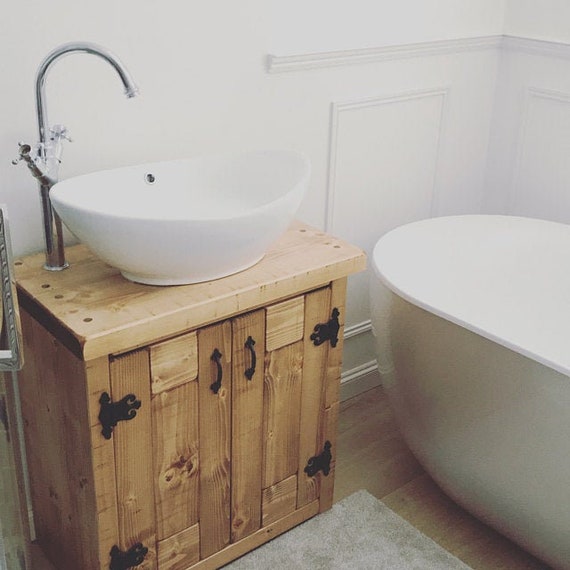The image showcases a corner of a sleek, modern bathroom characterized by its clean white walls and minimalist design. On the left side, there is a white ceramic basin style sink perched on a light-colored wooden cabinet, which features black hinges and doorknobs on its double doors. The sink boasts a chrome faucet, further emphasizing the contemporary aesthetic. To the right, part of a smooth, modern bathtub faces toward the corner of the room. The flooring beneath is hardwood, with a simple gray rug placed near the tub for stepping out. Overall, the bathroom exudes a sense of simplicity and modern functionality.